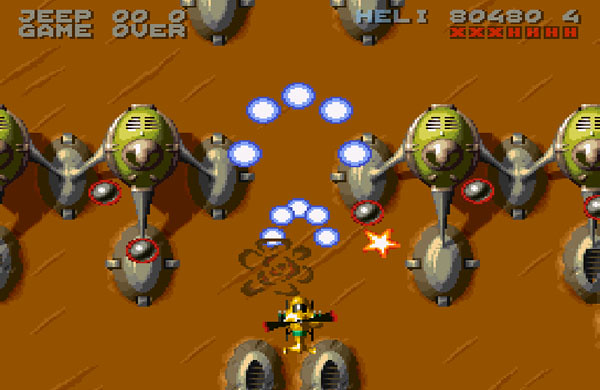This image is a screenshot from an old-school arcade game, presented with a top-down perspective. The background features a brown, desert-like terrain marked by diagonal dashes, suggesting sand. In the lower section of the image, two oval-shaped grey structures with grates are visible. Above these, a small yellow helicopter equipped with black and red rotors hovers. To its upper left, there’s a grey outline resembling either a flower or an explosion. Nearby, two semicircles of radiant white circles outlined in blue add to the scene’s mysterious atmosphere.

Dominating the central area are four structures, each composed of three metallic legs placed in a tripod formation, which support green ovals featuring ventilation slits. These complex constructs lend an industrial or sci-fi feel to the environment. Notably, text in the top-left corner reads "Jeep 000 Game Over" in grey. Similarly, the top-right corner displays "Heli 80,480" along with three red X's and three red H's beneath it, likely indicating player status or lives remaining in the game.